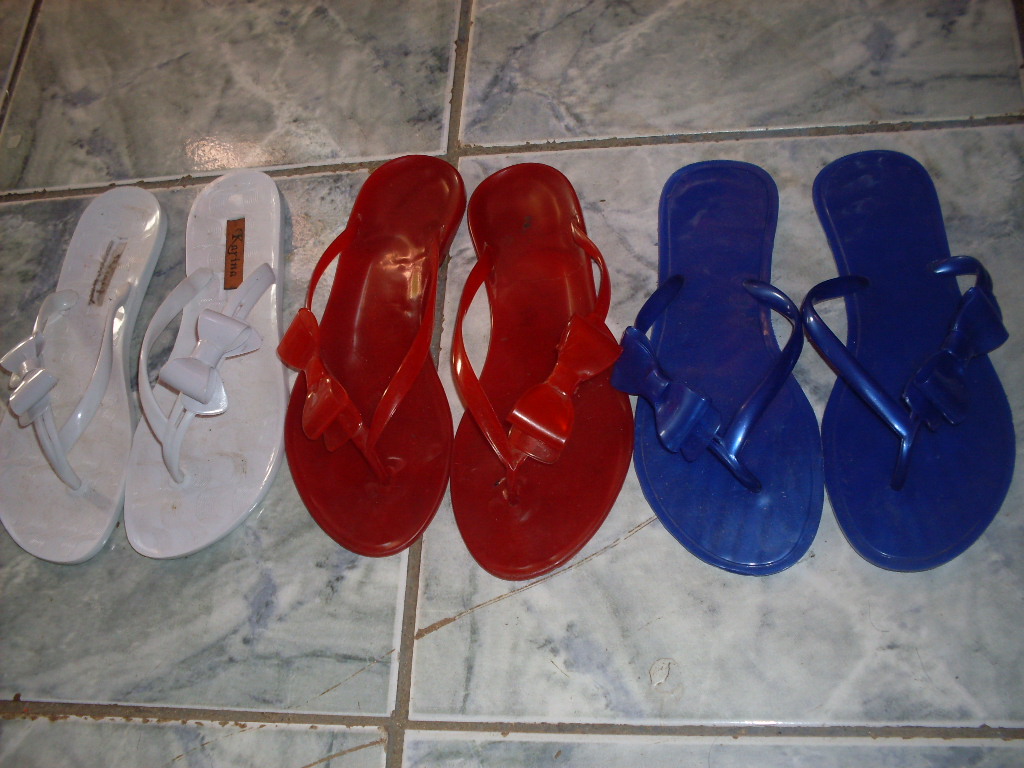This image captures a neat arrangement of three pairs of flip-flops positioned on an elegant, marble-tiled floor. The flooring features a grid of large, grey and white marbled tiles encased in sandy-colored grout, lending it a sophisticated appearance. From left to right, the flip-flops are white, red, and blue. Each pair is adorned with shiny, fancy bows on the thong straps, adding a touch of charm. The white pair, located on the left, has some writing on the heel, partly faded. All flip-flops are aligned facing downward, taking up more than half of the photo's frame. The overall perspective is from directly above, providing a close-up view of the scene.